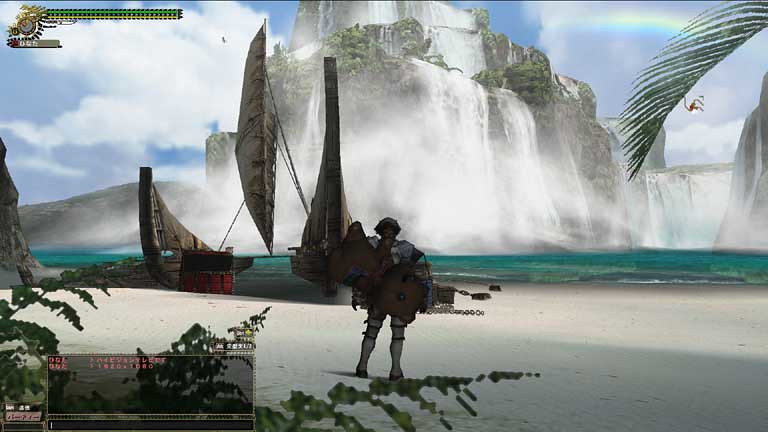The image is a digital screenshot from a video game, depicting a scene with a silhouetted character standing on a sandy beach. The character, potentially a man or woman, is outfitted in military-style gear, including a hat and a shield on their back, while also carrying a large backpack. This figure faces away from the viewer, obscuring their face. The landscape behind features a dilapidated boat composed of a larger rowing boat and a smaller one connected by a sail and a piece of wood.

The background is dominated by a towering mountain from which multiple waterfalls cascade down into clear water below. The sky above is a vivid blue with white clouds scattered across it. In the top left corner of the screen, a green and yellow health bar from the game’s user interface is visible, while in the bottom left, a chat box with a typing indicator shaped like an owl can be seen. The graphics are somewhat pixelated, indicating the game might have an older or stylized visual aesthetic.